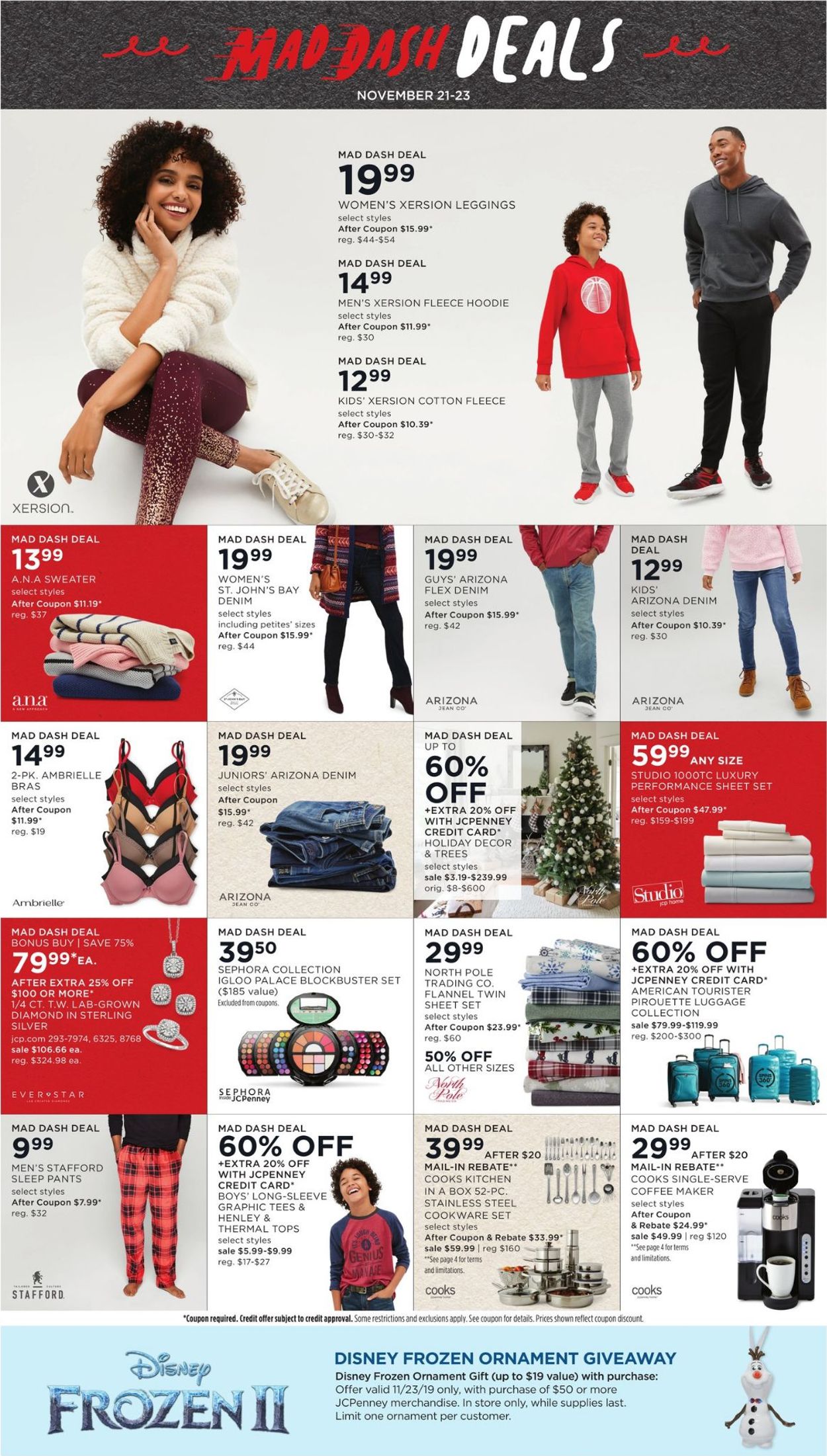The image is an advertisement for a "Mad Dash Deals" promotion. Set against a light blue background, the top of the advertisement features a black bar with dynamic red squiggles resembling movement. Bold red text that appears to be rushing says "Mad Dash," followed by "Deals" in white text. Below this, in small white text, the dates "November 21-23" are displayed.

In the first featured box, there is a woman dressed in a white fleece sweater and purple leggings with white spots. She appears to be relaxed and potentially shopping. Next to her, text highlights a "Mad Dash Deal" priced at $19.99, along with additional prices of $14.99 and $12.99 in smaller text. To her right, a man is wearing a gray hoodie, black pants, and black and red shoes, while a child beside him is dressed in a red hoodie, gray sweatpants, and red shoes. All three individuals are Black.

Below them, additional sales boxes are organized in rows:
- Top Left: Clothes, a skirt, jeans, and women's jeans.
- Second Row: Bras, jeans, a Christmas tree, and towels.
- Third Row: Diamond rings, necklaces, a makeup box, towels, and luggage.
- Last Row: Pajama pants, shirts, cookware, and a cooking pot.

Each item has a corresponding price listed.

At the bottom of the advertisement, a bar announces a "Disney Frozen 2" ornament giveaway. An image of an Olaf ornament from the movie "Frozen" is included, accompanied by some additional text.